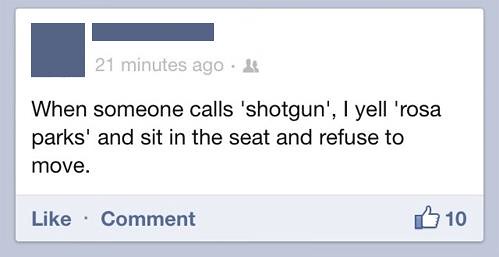This image is a screenshot of a social media post framed by a light blue border, featuring an obscured name and profile picture. The time stamp indicates it was posted 21 minutes ago. The post, hosted on a public profile, reads in black text, "When someone calls shotgun, I yell Rosa Parks and sit in the seat and refuse to move." Below the text, there are like and comment buttons in blue, accompanied by a thumbs-up symbol indicating the post has received 10 likes. The screenshot appears on a bluish background, highlighting the content against the white space of the display.